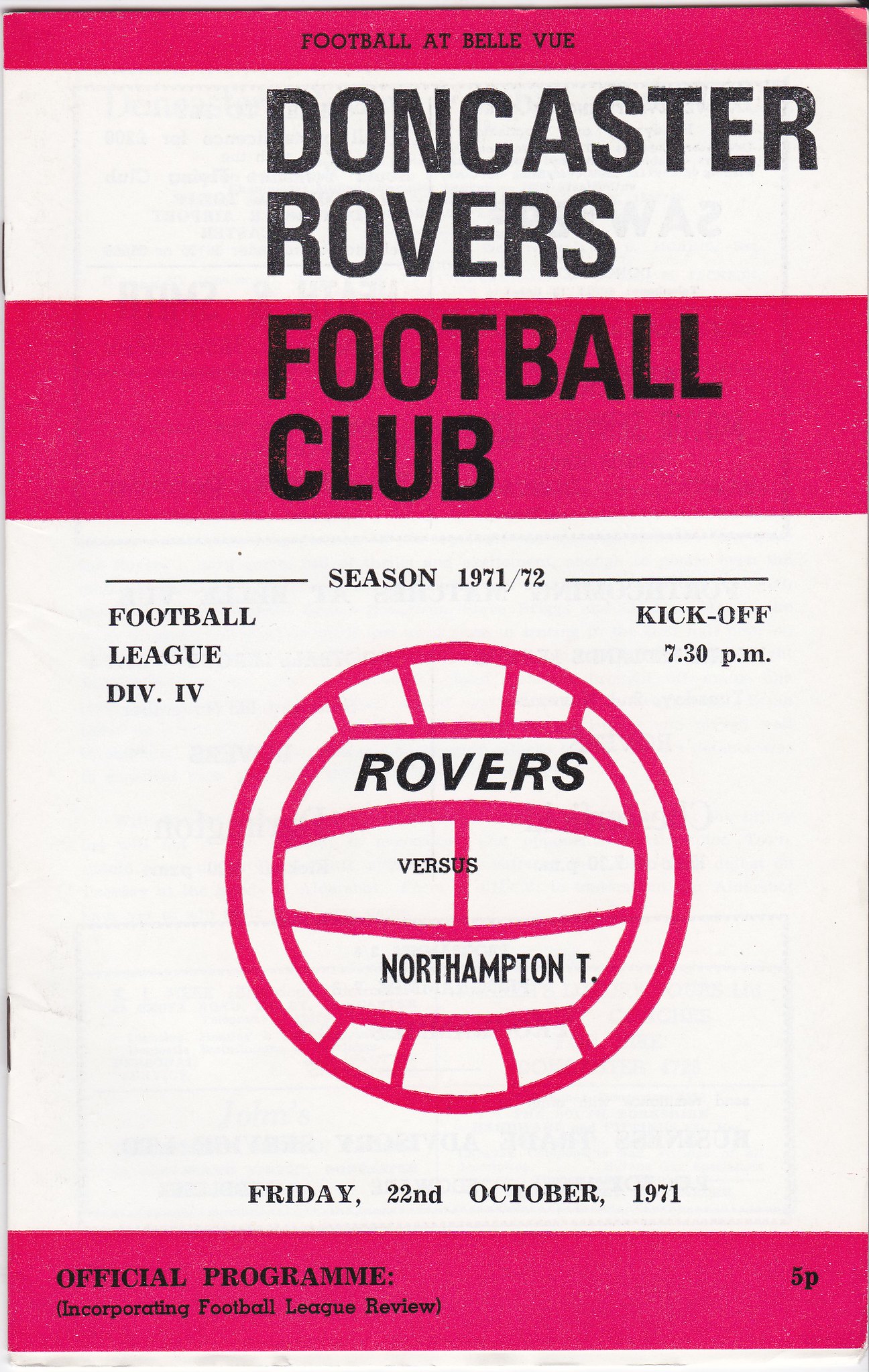The image is of a vintage football club program, specifically for the Season 1971-72, featuring a match between the Doncaster Rovers and Northampton Town, scheduled for Friday, 22nd October 1971, with kickoff at 7:30 p.m. The cover is designed with prominent pink sections at the top and bottom. At the top, within a wide pink band, it states "Football at Bellevue" and "Football Club" in black lettering. Central to the design is a large white area that displays the season "1971-72" and a football icon, which we would call a soccer ball in the U.S., with "Rovers vs. Northampton T" across it. On the left of this central section, there's "Football League Division IV" (with the four in Roman numerals), and on the right, the kickoff time. Below the football icon, the date "Friday, 22nd October, 1971" is clearly printed. The bottom pink band declares it as the "Official Program," which includes the "Football League Review" and is priced at 5 pence.